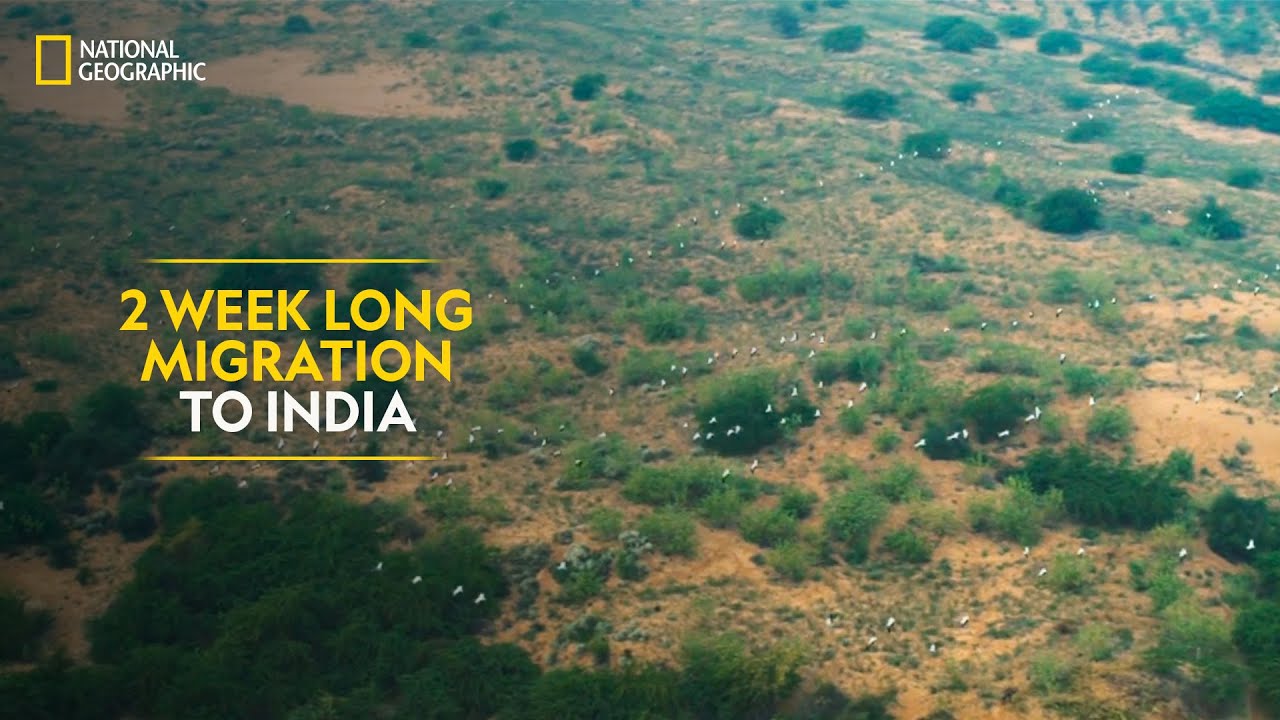The image is a still frame from a video, possibly a thumbnail, and features an outdoor scene in landscape layout, taken from an aerial perspective. It showcases a vast, barren area with varying shades of brownish-tan dirt interspersed with greenery from sparse grass, bushes, and small trees. The terrain suggests a Savannah or Saharan landscape, with light vegetation spread across the scene. In the image's upper left corner, the National Geographic logo, consisting of a small vertical rectangle with a yellow border and white text in two lines reading "NATIONAL GEOGRAPHIC," stands out. On the middle left side, there are two horizontal yellow bars with text in between them that fades to transparent towards the edges. The text reads "TWO WEEK LONG MIGRATION," in yellow, and "TO INDIA" in white, all in capital letters. There are no people visible in the image, and it includes what appears to be a flock of small white birds flying over the landscape, adding to the sense of a sweeping, natural scene.